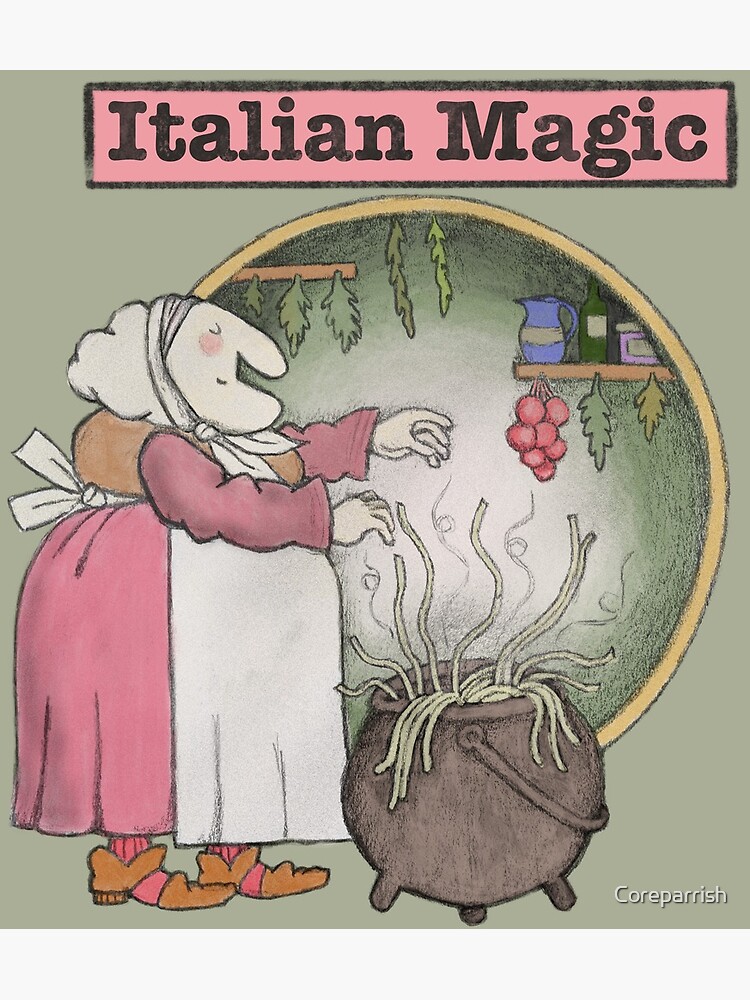The image is a detailed cartoon drawing titled "Italian Magic," written in black on a pink strip at the top, surrounded by a black border. It features Strega Nona, a beloved character from a children's book, known for her magic pasta pot that can produce endless amounts of spaghetti. Strega Nona is depicted as an elderly woman with a long nose and chin, a line for a mouth, a curved line for an eye, and a blush on her cheek. She wears a pink and orange dress with a white apron and a white handkerchief wrapped around her head. She also has pink socks and orange shoes. 

In front of her is a large brown pot with spaghetti noodles rising towards her outstretched hands, evoking a sense of magical cooking. Surrounding the scene are various ingredients and cooking items, including jars, bottles, red radishes, green herbs, and berries, all arranged on shelves and hanging from the background. The overall setting has elements that resemble a kitchen infused with a touch of magic, enhanced by the warm and inviting color scheme of pinks, oranges, and browns.